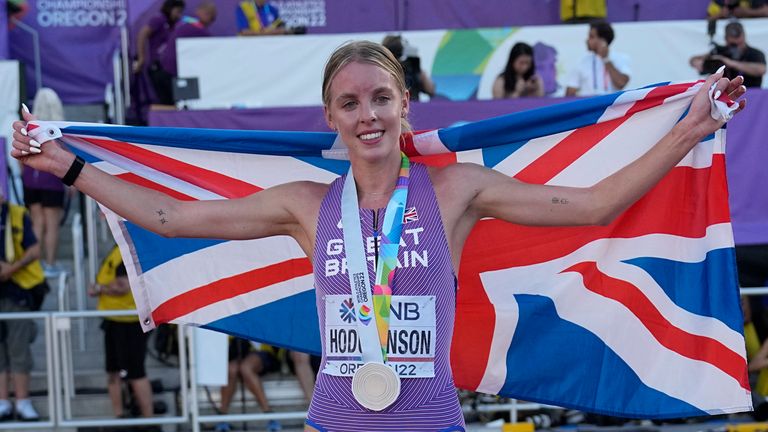The image captures a female athlete in the midst of a competition, possibly track and field. She is standing proudly at the center, holding a British flag with her arms outstretched. The flag, characterized by its red, white, and blue pattern, drapes behind her like a cape. The athlete is Caucasian with dirty blonde hair pulled back. She is smiling broadly, showing her bright white teeth and has noticeable red lips. Her sleeveless, tight purple tank top features thin white stripes and has "GREAT BRITAIN" written across the chest, although partially obscured by a lanyard. The lanyard, colorful with shades of blue, green, orange, pink, and various greens, holds a white circular medal, likely indicating she has placed in the event. Below "GREAT BRITAIN" on her uniform, the name "Hodgson" and her race number are also partly visible. The background reveals faint, out-of-focus details, showing spectators, event staff, possibly championship signage, and rails. The signage appears dark purple, and mentions "Championship, Oregon." The image captures a moment of triumph and national pride at a notable sporting event.